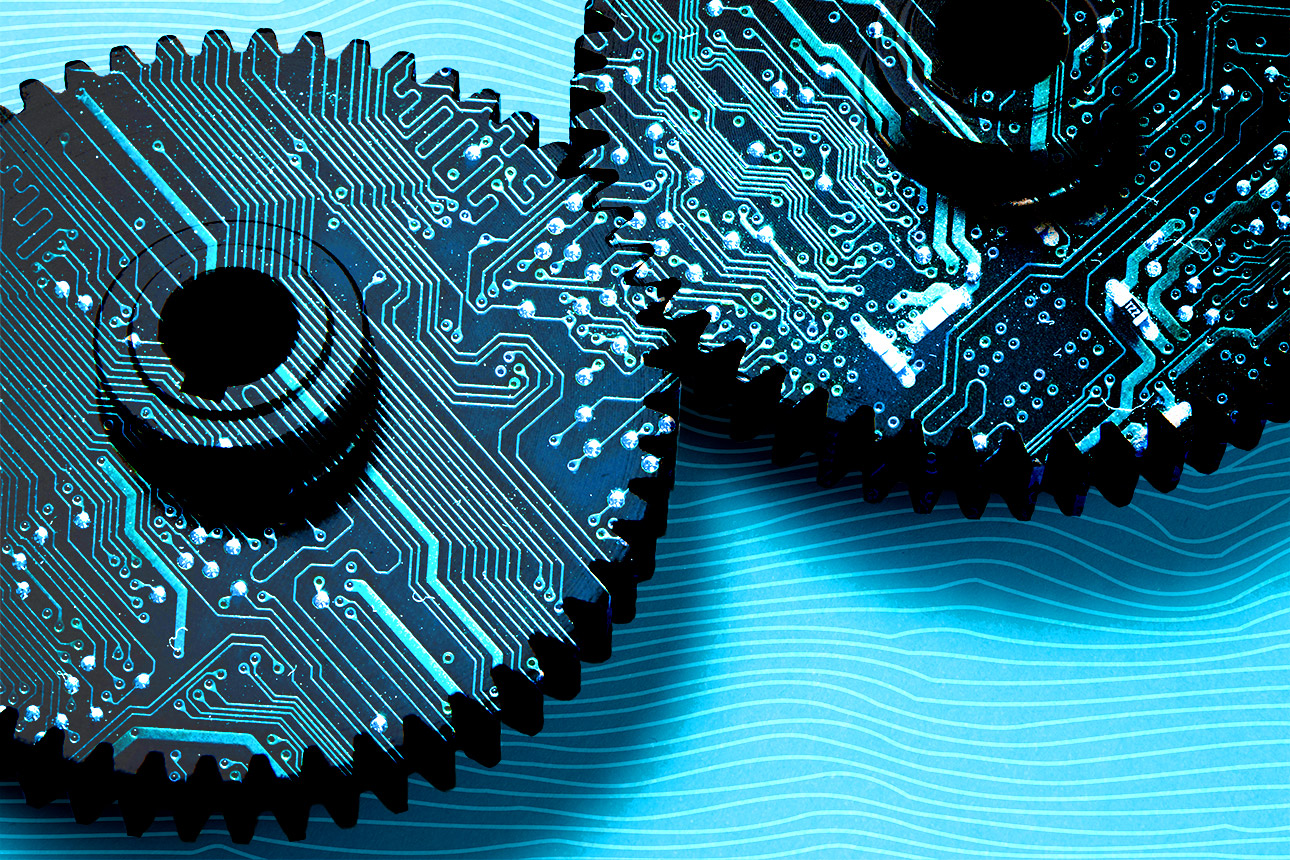This image captures two partially visible interconnected gears with interlocking teeth, positioned diagonally from each other on a blue background adorned with white wavy lines. The gears exhibit intricate circuitry, with light blue circuit lines reminiscent of those on a circuit board, winding through their metallic surfaces. Both gears feature two small protrusions in their centers. The left gear sits slightly lower than the right, and both cast shadows that vary the blue background's hue. The overall composition hints at a horizontal rectangular format, with the gears' circuitry and the white wavy lines creating a vivid, technical aesthetic.